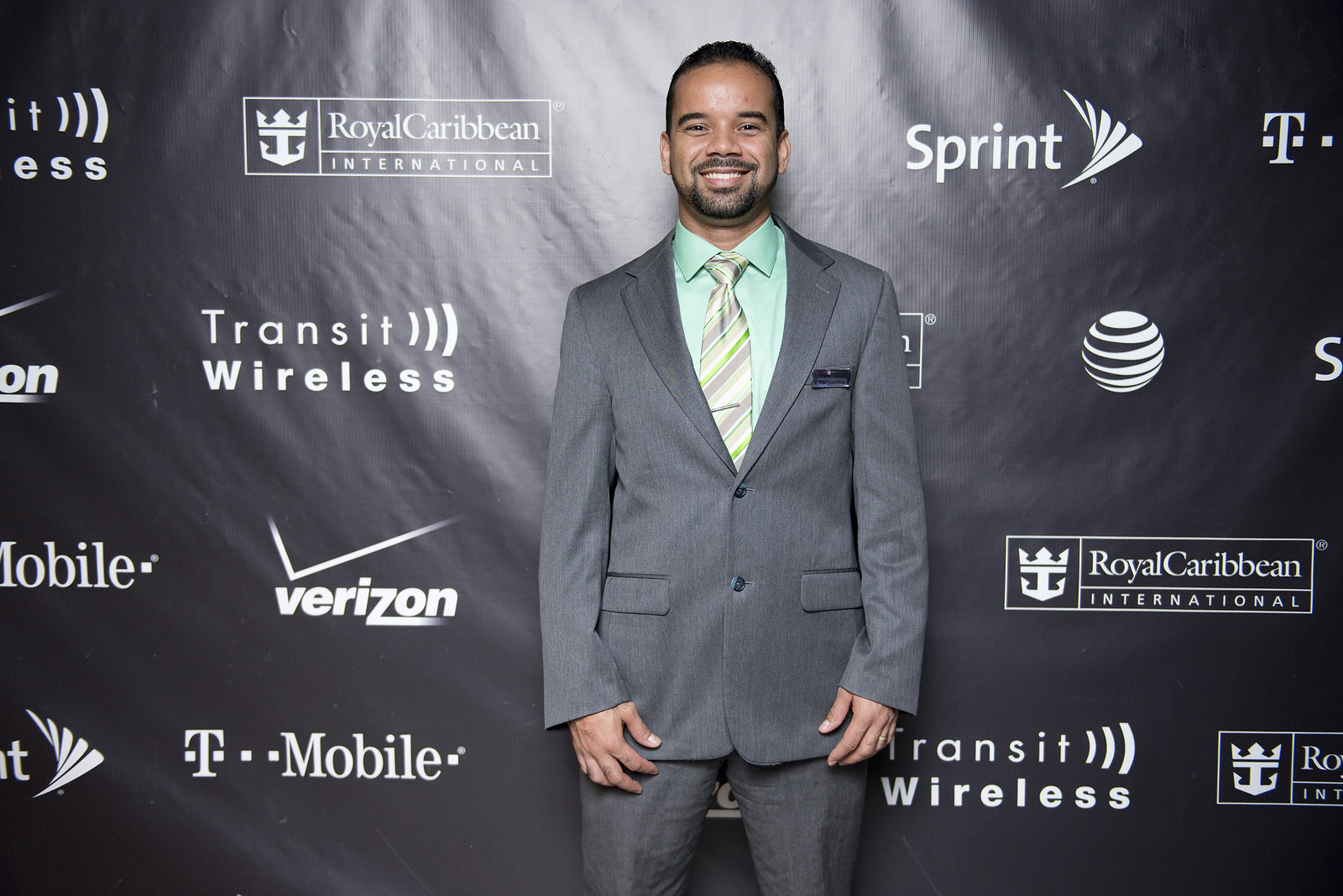A man with dark brown skin, a mustache, and a short beard stands confidently in front of a black plastic-covered wall adorned with white brand names and logos such as Royal Caribbean, Sprint, Transit Wireless, Verizon, T-Mobile, and AT&T. He's dressed in a sharp grey two-piece suit, complemented by a light green button-down shirt and a striped tie featuring grey, yellow, green, and light purple hues. A black name tag is clipped to his attire, though its text is not legible. He smiles slightly as he stands with his hands at his sides, exuding a polished and professional demeanor.